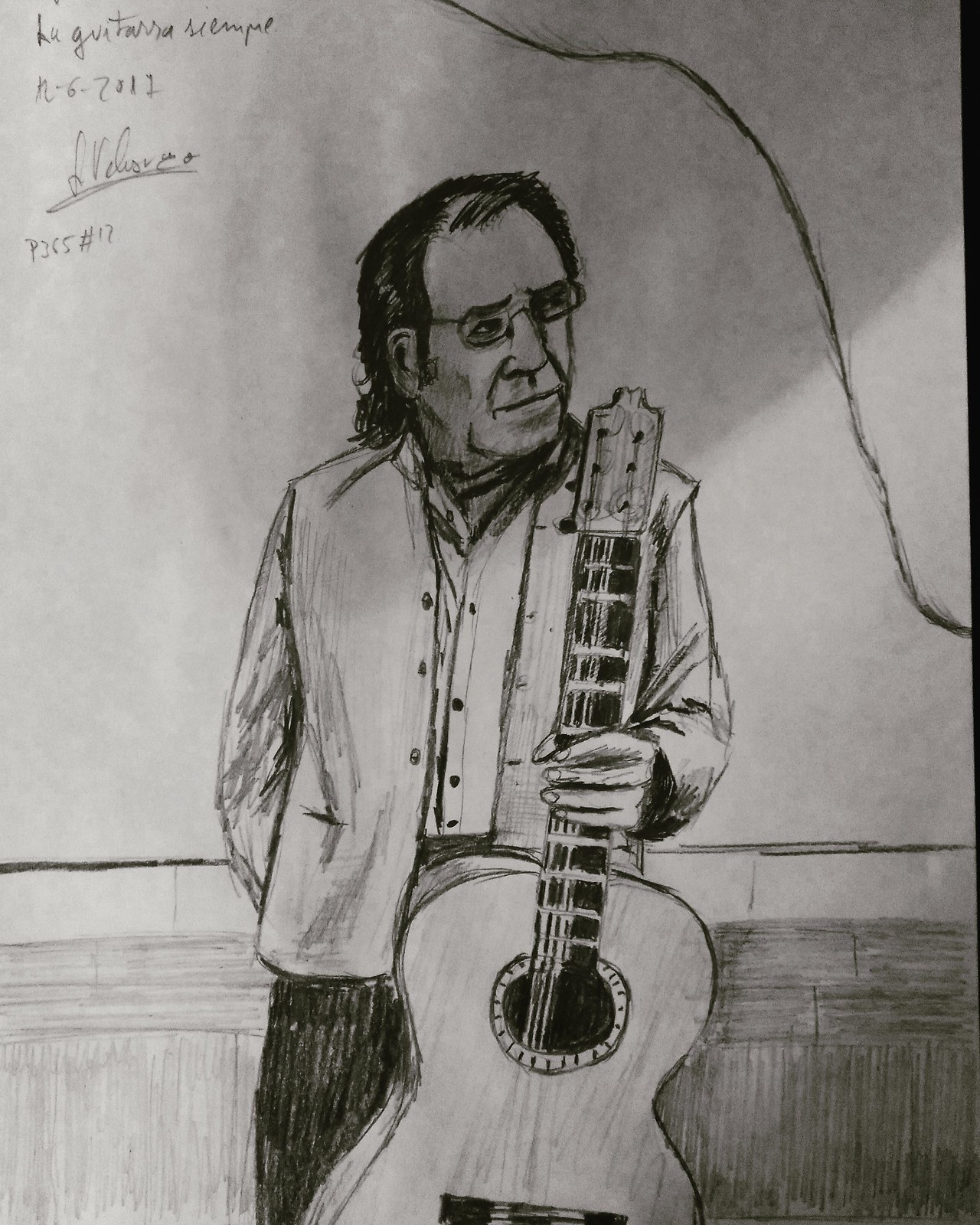This is a detailed pencil drawing of an older man holding an acoustic guitar. The artwork is on sketchbook paper, with part of the entire page visible. In the upper left corner, there's some text that reads “La Guitara Siempre” and is dated 12-6-2017 (or possibly 2-6-2012, according to another caption). The man, facing towards the right, is balding on top with a few strands combed over; the longer hair at the back forms a mullet. He wears rectangular eyeglasses and displays age lines around his mouth, nose, and chin. He is dressed in a long-sleeved button-up shirt, unbuttoned at the top, layered with a vest, and dark-colored jeans. His right hand holds the neck of the guitar, while his left arm is positioned behind his back. He appears to lean against a wall, which is depicted with a distinctive large crack extending from the top of the page down to the right. The wall is wooden at the bottom and lighter at the top, possibly indicating a stage setting behind him.